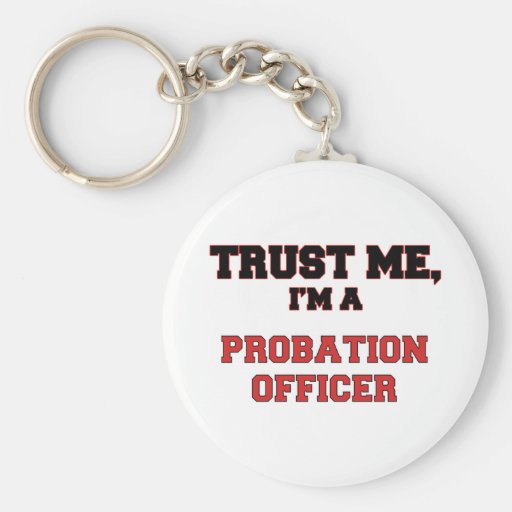The image showcases a keyring against a stark white background with a faint shadow cast around it. The main element of the keyring is a round, glossy white medallion, adorned with bold text that has a strong, authoritative feel akin to what you might find on official government equipment. The text on the medallion reads "TRUST ME I'M A" in black, capital letters, followed by "PROBATION OFFICER" in striking red capital letters. The medallion is connected to a bronze chain comprised of five loops, which in turn attaches to a larger bronze ring designed to hold keys. The overall presentation is straightforward, emphasizing the keyring's official and bold design elements.